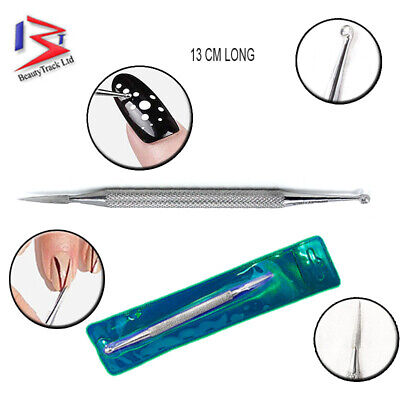This is a detailed promotional image for a versatile nail styling tool by Beauty Track Limited. The upper left-hand corner features their logo, a sideways red "M" with two blue lines extending upward, accompanied by the name in black font. The focal point is a 13-centimeter-long, silver beauty instrument with a round, hard end on one side and a needle-like brush tip on the other. It includes a textured grip in the middle for ease of use. The right side of the image presents two close-up, circled views of the tool's ends, highlighting its precision. Additional smaller images showcase its applications: the tool is shown in a green sterile plastic pack, painting fine lines and creating intricate nail art such as white polka dots on black polish and brown branch-like designs on clear polish. The tool is also depicted in use for bedazzling and detailed nail painting, demonstrating its multifunctionality in nail art decoration.